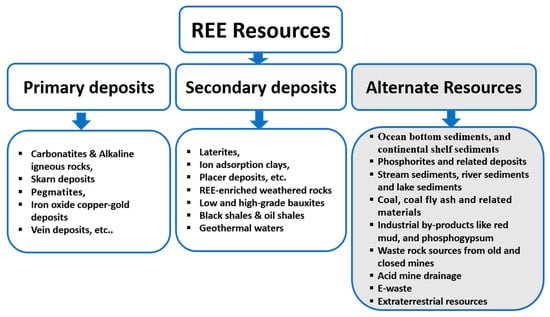The image depicts a detailed diagram with a white background, bounded by a series of blue-bordered, rounded rectangles and squares. At the top of the diagram, the largest box is labeled "REE Resources" in black text. From this top box, a blue arrow points downward to a second row of three columns, each representing different types of deposits. 

The first column is labeled "Primary Deposits," listing types such as carbonatites, alkaline igneous rocks, scarn deposits, pegmatites, iron-oxide copper gold deposits, and vein deposits. 

The second column is labeled "Secondary Deposits," including laterites, ion-adsorption clays, placer deposits, REE-enriched weathered rocks, low and high-grade bauxites, black shales, oil shales, and geothermal waters. 

The third column, marked as "Alternate Resources," is the largest column and is highlighted in gray. This section includes a more extensive list, such as ocean bottom sediments, continental shelf sediments, phosphorites and related deposits, stream sediments, river sediments, lake sediments, coal, coal fly ash and related materials, industrial byproducts like red mud and phosphogypsum, waste rock sources from old and closed mines, acid mine drainage, e-waste, and even extraterrestrial resources. 

Below each main category, more specific details and lists are provided, with blue arrows guiding the flow from the general resource types down to specific deposit examples.